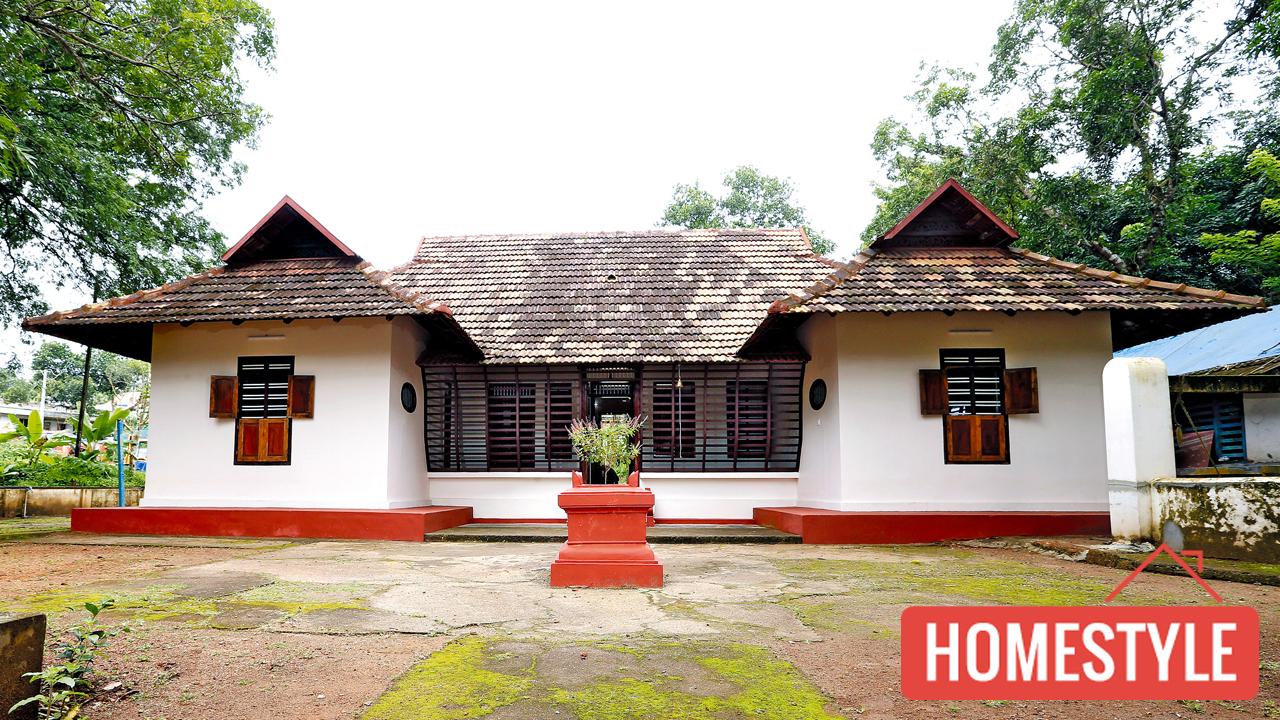The image showcases a picturesque house displaying traditional Eastern Asian architectural elements, possibly from Thailand or India, surrounded by lush and verdant greenery hinting at a humid, tropical setting. The house features striking white exterior walls with vivid red borders along the base, which contrasts beautifully with the earthy, worn brown roof tiles. The central focus of the image is a raised red platform, possibly holding a garden bed or a Tulsi plant, indicative of Indian design. The structure boasts wooden window flaps—two of which are open at the top, offering glimpses into the interior, while the lower ones remain closed. The roof has a tiered design, with the main roof descending into smaller peaked sections on either side, covered in light white and gray tiles, with the side sections having a more brownish hue. The front lawn is a rustic mix of dirt and green patches, accentuating the natural aesthetic of the scene. This image, likely sourced from an accommodation website, is taken during daylight, as seen from the clear white sky, enhancing the charm of the house. At the bottom right of the picture, against a red background, the text "Home Style" is prominently displayed in white print.